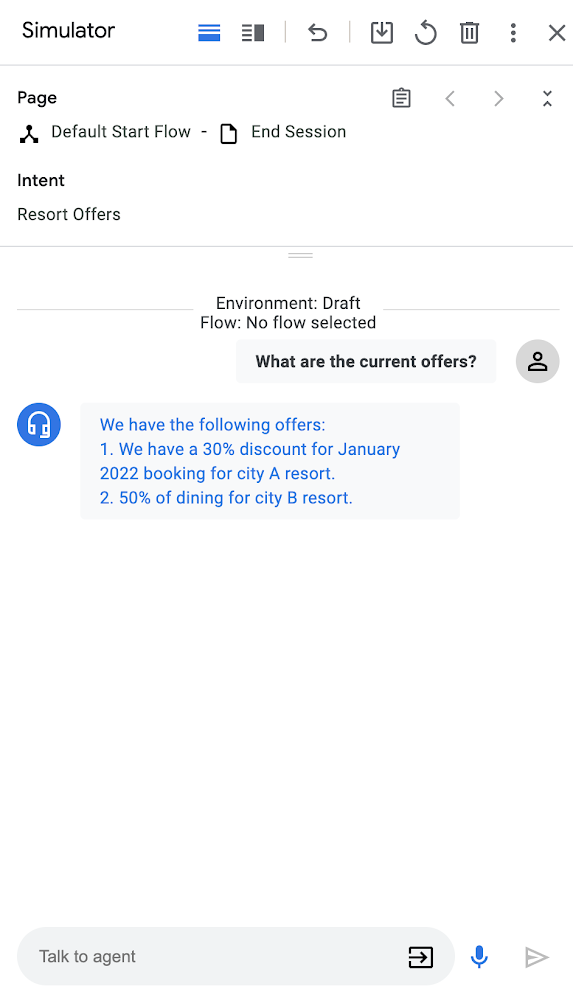This is a detailed screenshot of what appears to be the settings or chat interface of a web application, possibly a simulator. The background is white. In the upper left corner, in black font, the word "Simulator" is displayed. To the right, there are several icons arranged horizontally, including three blue lines, four black lines with a black rectangle beside them, a return arrow, a download button, a refresh arrow, a trash can icon, three vertical gray dots, and an X icon.

A black line runs below these icons. The word "Page" appears at the top. To its right, there is an icon resembling a check clipboard, followed by a left arrow and a right arrow. Beneath these elements, the text "default start flow -" is displayed, accompanied by an icon of a page with the label "End Session" next to it. Directly below, the word "Intent" is shown, followed by the text "Resort Offers."

Further down, there are two gray lines separated by some space. Centrally positioned on the lower gray line is the text "Environment: draft flow - No flow selected."

Below this section, a chat bubble interface is visible. A user-query bubble reads, "What are the current offers?" The response, displayed in blue font, states, "We have the following offers: 1. We have a 30% discount for January."